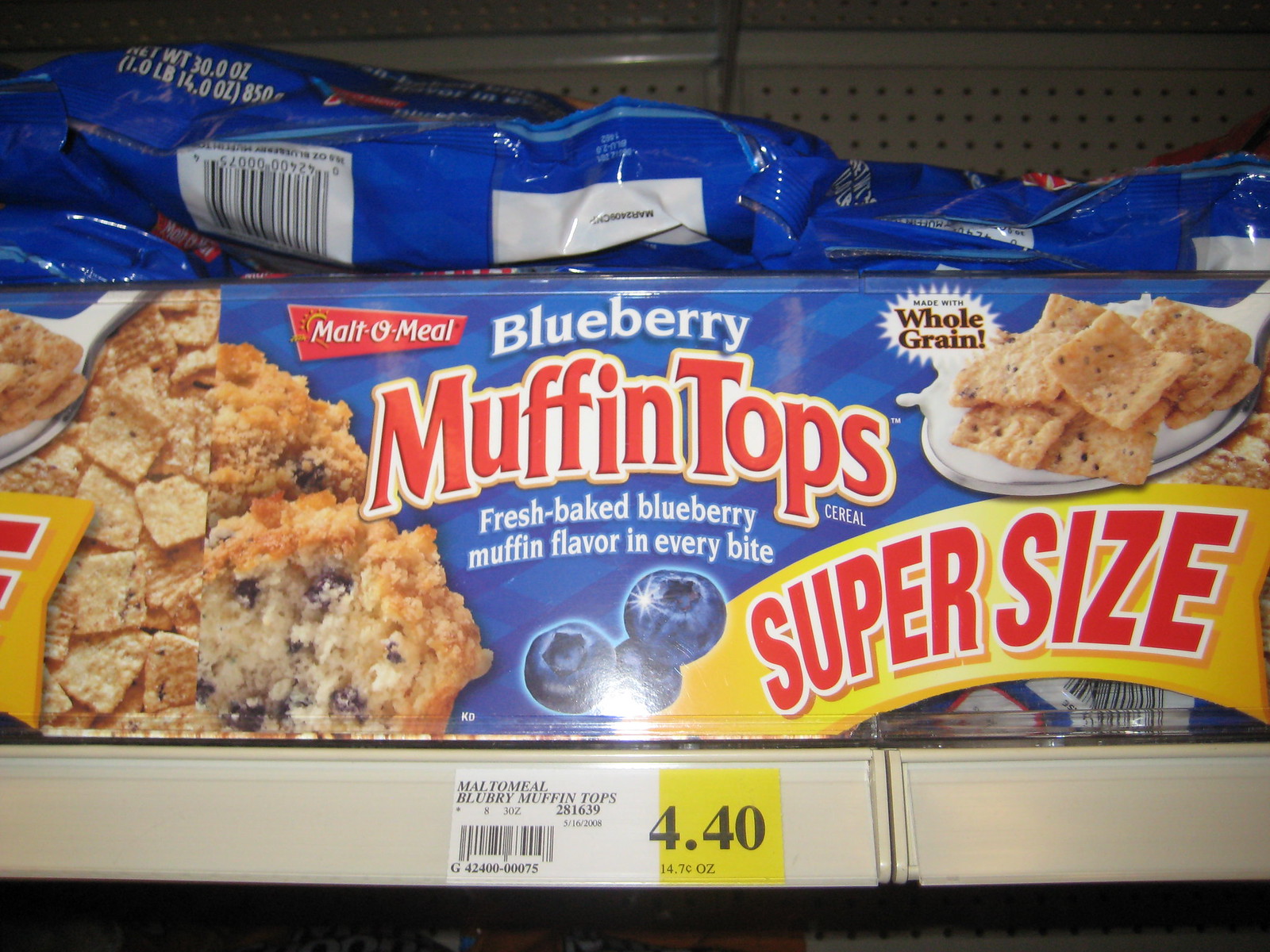The image is a color snapshot photograph in a horizontal orientation, capturing a shelf in a grocery store. The shelf has a metal tag displaying the number '440' and provides details for the product "Malt-O-Meal Blueberry Muffin Tops," including a UPC symbol. Above the shelf, there are plastic laminate sections with banners running across the entire image from left to right, prominently featuring the text "Blueberry Muffin Tops Super Size." The banner illustrates various types of blueberry muffins, presenting them as if they were crackers on a spoon. The top of the shelf is lined with plastic packaging in vibrant colors, including blue, red, yellow, and light brown, which match the crumb topping of the muffins. Additionally, the labels underneath the shelf are light brown and yellow, adding to the visual appeal and cohesive branding of the display.